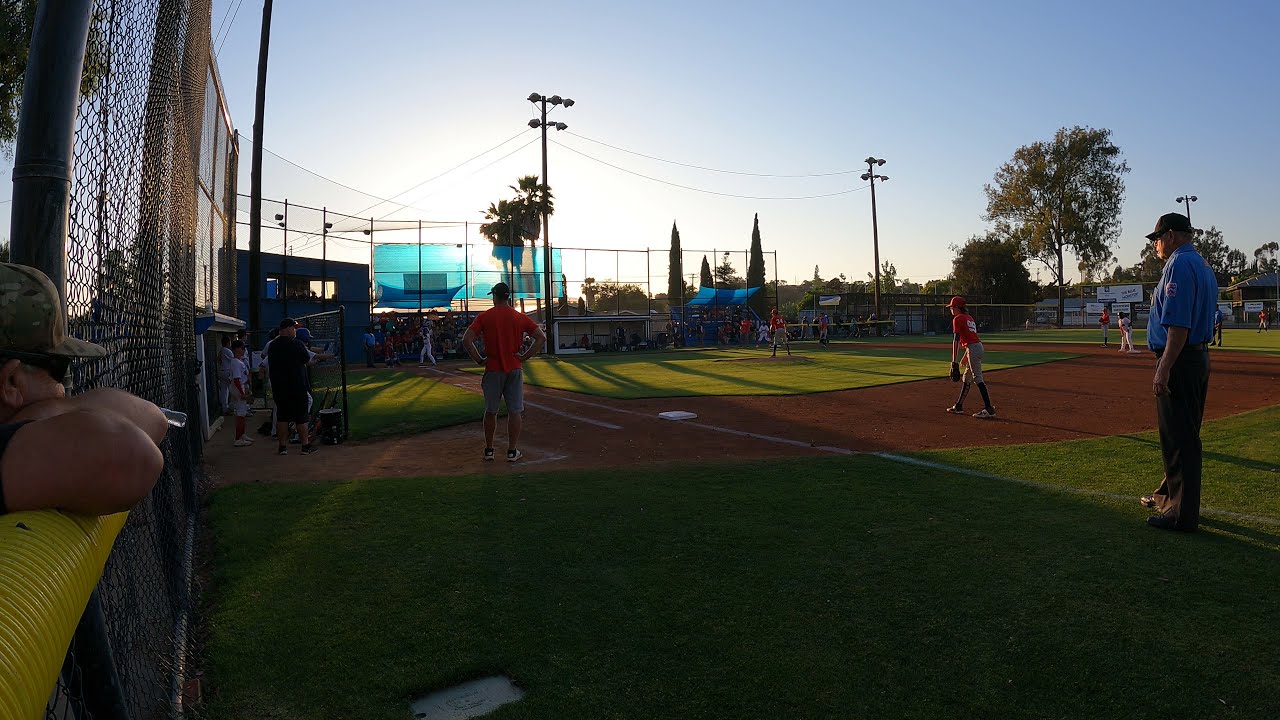The image captures a vibrant afternoon kids’ baseball game set on a well-maintained diamond. The scene is viewed from behind first base, where a spectator in a camo hat is leaning on a yellow barrier, closely watching the game. The field is lush with very green grass, and the background features numerous green trees, indicating a warm, likely summertime setting. The sun is setting low in the sky, casting dynamic lighting over the field.

The action centers around a player in white at bat, with their team's dugout visible on the left-hand side of the image. The red team is the fielding team, sporting red shirts, gray pants, and red hats. An umpire dressed in a blue shirt stands near first base. The backdrop of the image includes a big chain-link fence, large stadium lights on tall poles, and another field to the right. In the far end near third base, one can spot spectators enjoying the game. The suburban setting is underscored by the presence of houses in the distance, completing this dynamic, sunlit scene of a community baseball game.